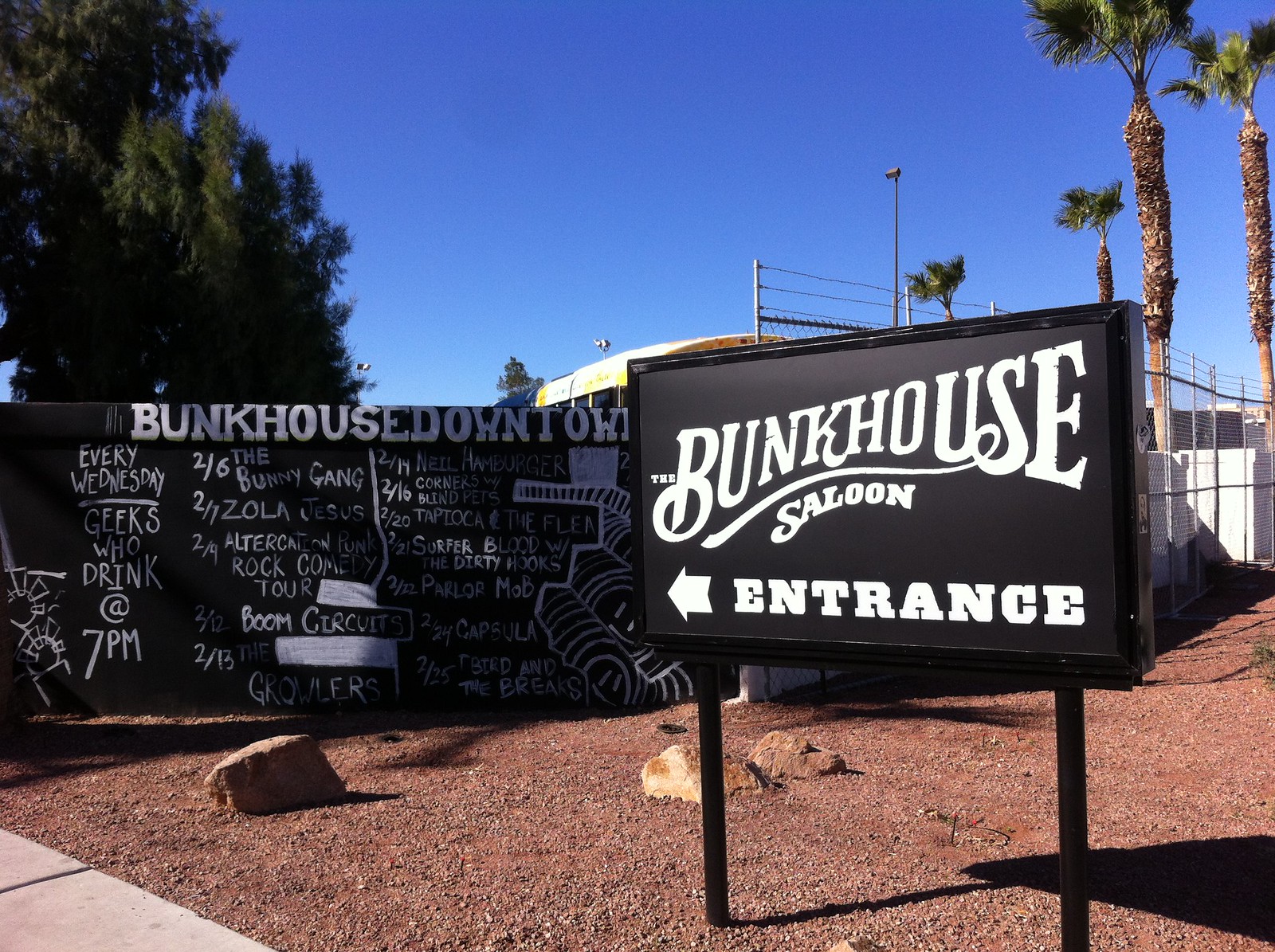This outdoor photograph features a prominently placed black sign with bold, white text reading "The Bunkhouse Saloon" and an arrow pointing left, indicating the entrance. To the left of this sign stands a stone wall adorned with various chalk-written announcements. The wall, labeled "Bunkhouse Downtown," displays a series of events: "Every Wednesday Geeks Who Drink at 7 p.m.," followed by scheduled performances including "2/6 The Bunny Gang," "2/7 Zola Jesus," "2/9 Altercation Punk Rock Comedy Tour," "2/12 Boom Circuits," and "2/13 The Growlers." The background reveals a mix of trees, including palm varieties, some fencing, a building, and even a school bus, creating a vibrant yet informal scene dominated by these informative signs.